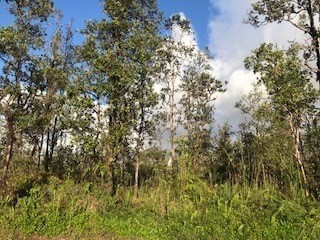The image depicts a small, low-quality rectangular landscape of a sparse, overgrown forest. In the foreground, there are patches of green grasses and shrubbery mingled with light orange and tan hues, suggesting a transition of seasons. The scene is dominated by numerous tall, slender trees whose narrow trunks vary in color, ranging from dark black and tanned brown to white. The trees, adorned with sparse, narrow leaves, extend upwards with their tops slightly cut off by the top edge of the image.

In the background, a clear blue sky occupies the top left corner, gradually giving way to a mass of white clouds or possibly smoke rising from the right-hand side, hinting at a potential distant forest fire, though no flames are visible. The setting feels remote and untouched, as suggested by the overgrown grasses, and the overall impression is of an unoccupied, quiet woodland with a hint of seasonal change.